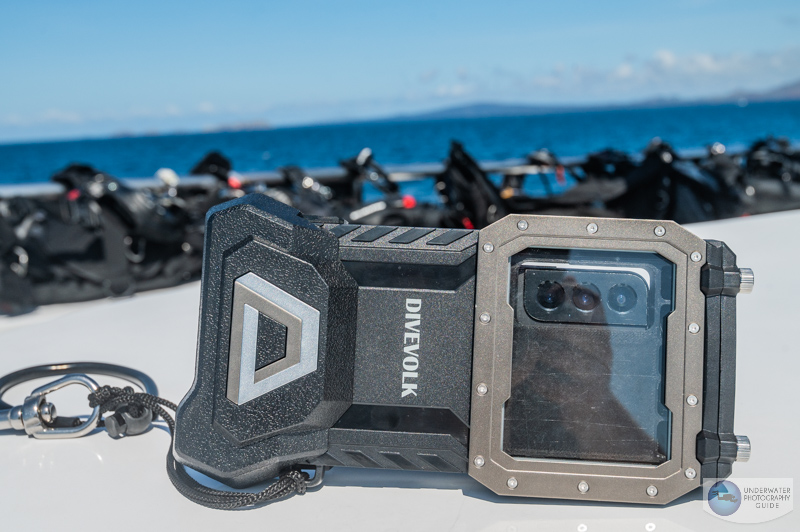In the picture, we see an electronic device, presumably a camera, resting on the white deck of a boat. This device is rectangular with a black plastic frame and features a clear, reflective screen on its right side, showcasing the surrounding environment. On the left side of the device, there is a black rope connected to a carabiner, likely for securing it. The device bears the name "DiveVolk" prominently in the center.

The brand logo, a white rectangle with a curve at the bottom and a dot, appears in the bottom right corner, labeled with "Underwater Photography Guide". The middle of the device also displays a prism-like logo resembling an optical illusion in grey and white. Additionally, three camera lenses are visible on the top right inside a protective case.

In the background, we see the bright blue sea and a blue sky above. Various pieces of black and silver gear are attached to a silver railing along the pier, enhancing the impression of a nautical setting.